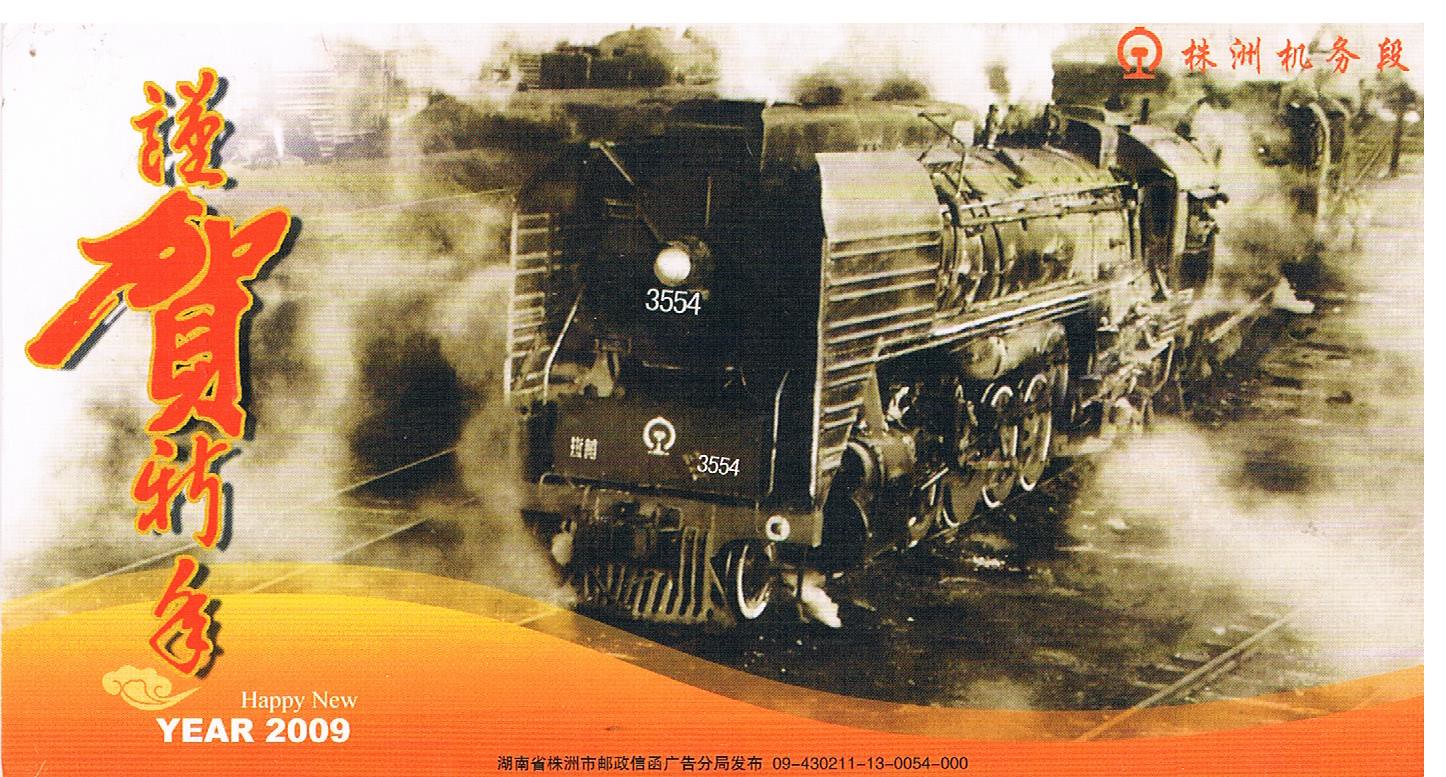The image is a detailed drawing of an old black-and-white locomotive, prominently labeled with the number 3554 on both its front and lower sections. The train, an archaic model, occupies three-quarters of the picture, primarily situated in the upper and center-right areas as it appears to progress forward. Visible wheels and attached train cars extend into the upper right background, providing additional context to the locomotive's path.

Overlaying the upper right corner of the image are six orange Asian characters, potentially Japanese or Chinese. Accompanying these symbols is a logo resembling either a lantern or an 'on' button. Additional Asian characters are also present on the left side of the image, stylized with a yellow outline and a black drop shadow. 

In the bottom left of the picture, "Happy New Year" is inscribed in white lettering, with "2009" displayed prominently beneath it. The entire text appears against a deep orange background. Further black Asian characters are centered along the bottom, next to a sequence of numbers: 0943021130054000. The detailed composition emphasizes a harmonious blend of the locomotive imagery with culturally significant symbols and text, celebrating the Happy New Year of 2009.